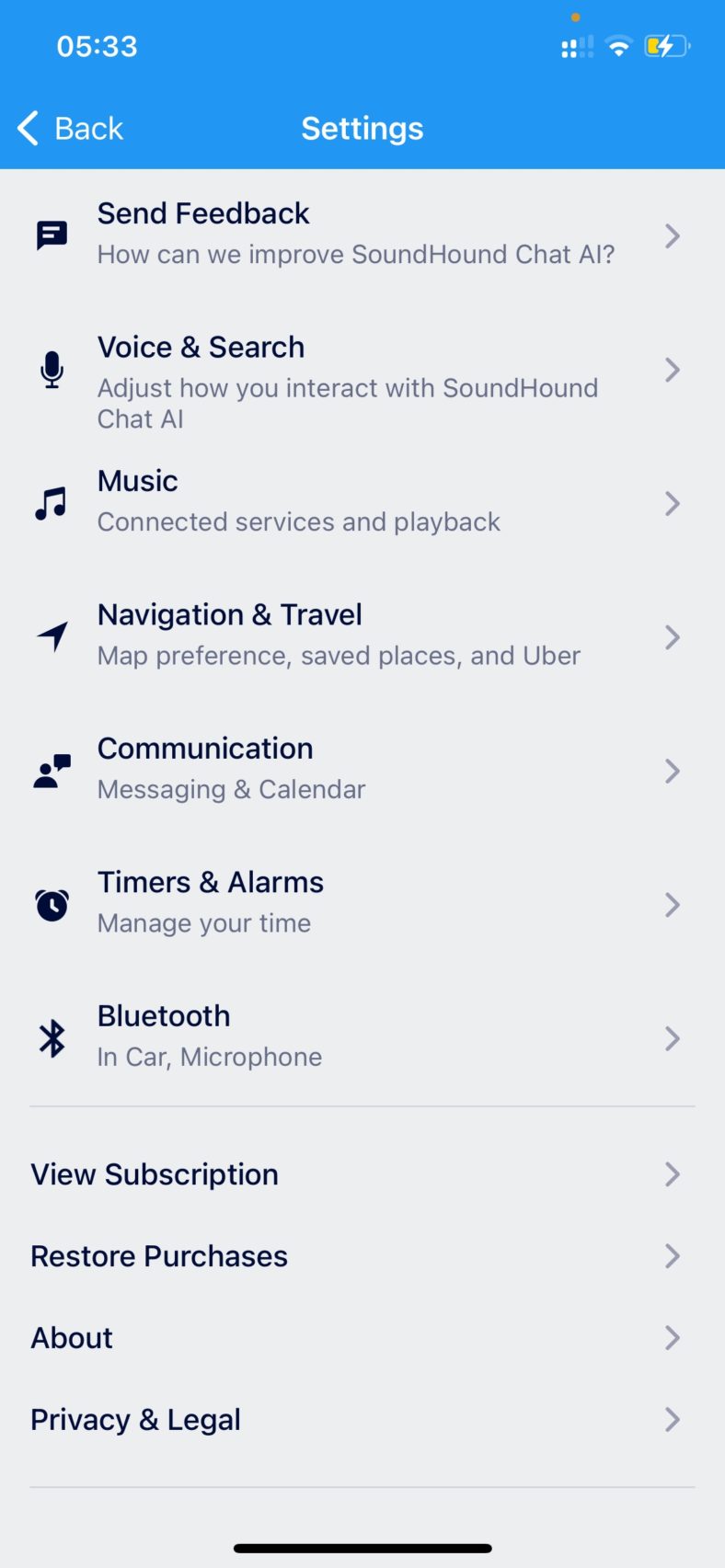The image depicts a smartphone screen showing the settings menu for the SoundHound Chat AI application. The status bar at the top displays a blue background, a "533" signal indicator, 2 out of 4 bars of cellular signal, 2 out of 3 bars for Wi-Fi signal, and a yellow battery icon with a lightning bolt inside, indicating charging status. 

Below the status bar, there is an option labeled "Send Feedback" followed by a prompt asking "How can we improve SoundHound Chat AI?" This prompt is part of the settings options available to customize the interaction with the SoundHound Chat AI. The settings categories include:

1. **Voice and Search**: Adjust preferences related to voice commands and search functionalities.
2. **Music and Connected Services**: Configure linked music services and playback customization.
3. **Navigation and Travel**: Set map preferences and integrate safe places and Uber.
4. **Communication**: Modify settings for messaging, calendar integration, timers, and alarms.
5. **Manager**: Manage time, Bluetooth connectivity, and car microphone settings.
6. **View Subscription and Restore Purchases**: Manage subscription details and restore previous purchases.
7. **About, Privacy, and Legal**: Access app information, privacy policies, and legal terms.

The screen background is gray, and the layout presents a clean and organized interface, facilitating easy navigation through various settings. There are a total of seven different options displayed on the screen.